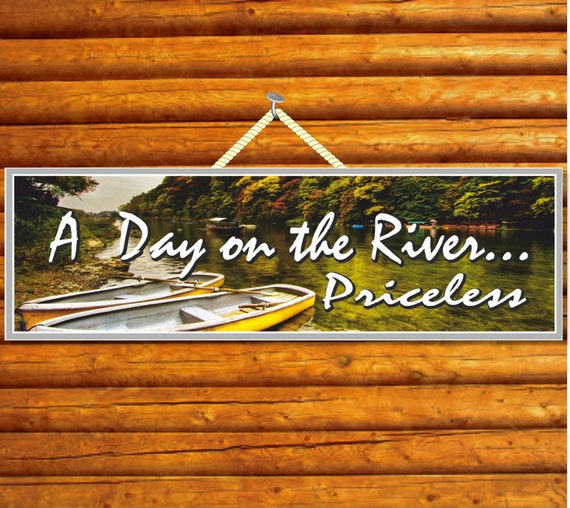The digital photograph captures a rustic wooden wall made up of brown logs, with a sign prominently displayed. The sign, framed in gray, features the text "A day on the river, priceless" in white lettering. This sign is anchored to the wall by a nail and set against a background that includes two yellow sailboats. These sailboats are pictured side by side, seemingly docked near a calm river. The serene setting hints at nature's tranquility with the presence of a distant forest, further enhancing the idyllic and priceless experience described by the sign. The overall color palette of the image includes shades of brown, yellow, white, and subtle hints of gray and orange.